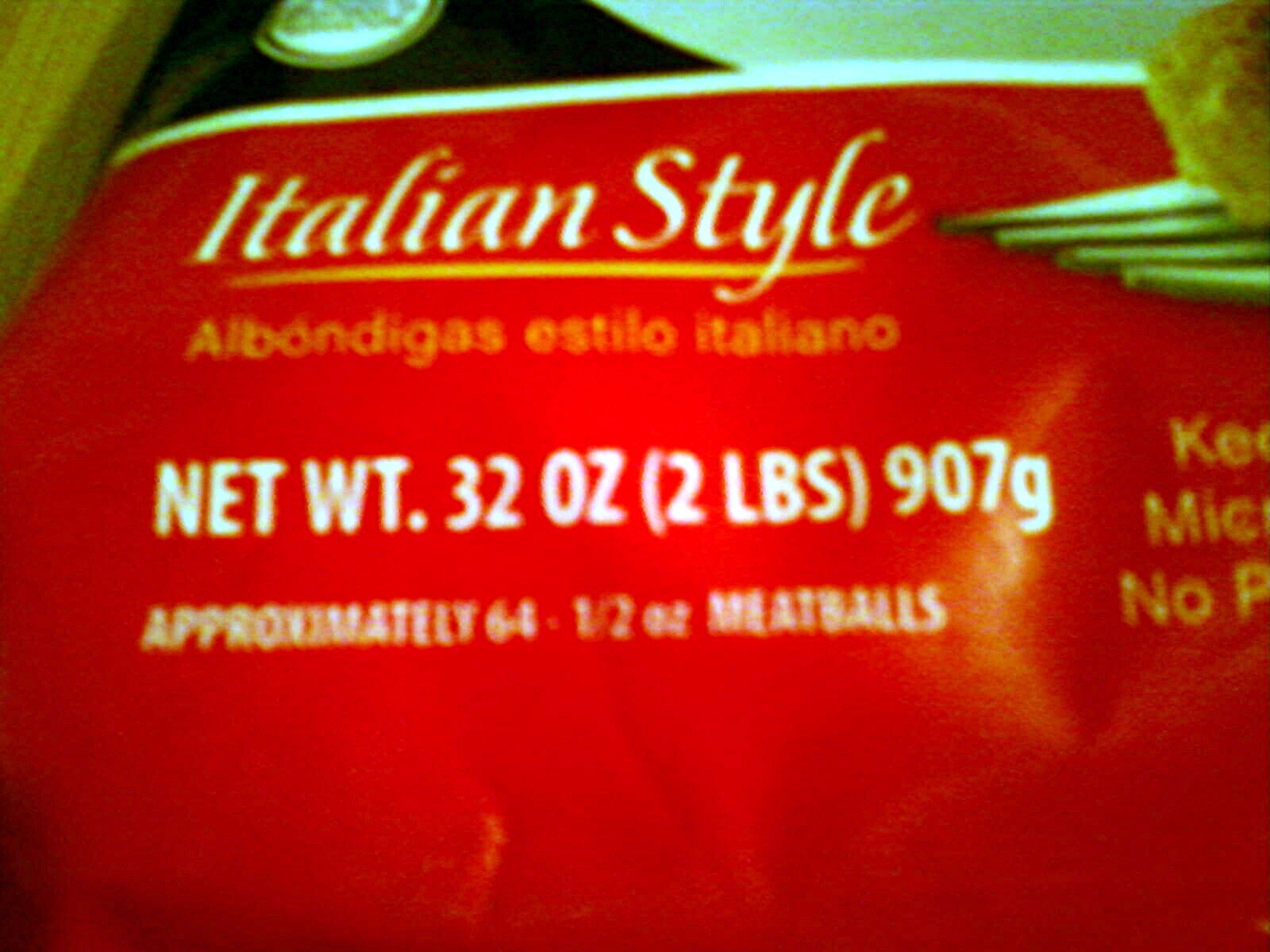The image depicts a label for an Italian-style product, though the exact nature of the product is indeterminate. The label prominently features a red banner across the top with the words "Italian-Style" written in white. Below this, a section of text in yellow displays Italian words, enhancing the authentic feel of the product. The label also specifies that the net weight is 32 ounces, equivalent to 2 pounds or 907 grams. It mentions that the product is sufficient for making approximately forty-six Italian-style meatballs, suggesting it is likely a seasoning mix or ingredient intended to be blended with meat to create traditional Italian meatballs. The overall design and language aim to evoke an authentic Italian culinary experience.